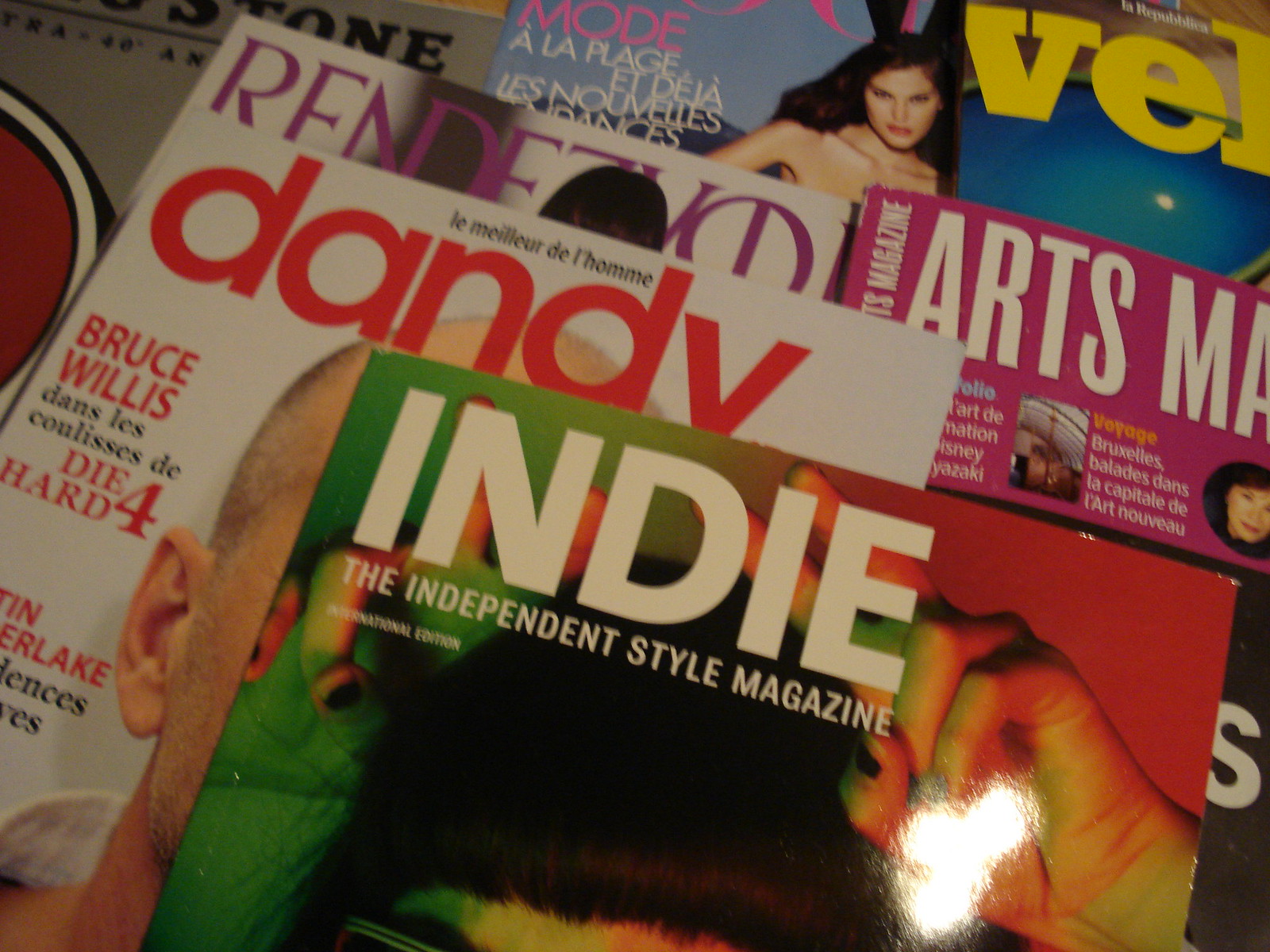This aerial view highlights a wide rectangular stack of overlapping magazines, making it difficult to discern the surface they rest on. Prominently featured at the bottom of the image is a tilted magazine titled "Indy, the independent style magazine, international edition," displayed in bright white font. Under green and red lighting, the magazine cover shows a woman with black hair and bangs, her hands raised above her head in double peace signs. Slightly obscured behind it, yet visible, is another magazine with a white background named "Dandy," written in red font. The visible part of its cover mentions "Bruce Willis, Die Hard 4," though the exact clarity on the image may vary. The overlapping arrangement reveals portions of other magazines: "Renzezo" in purple letters, a pink magazine hinting at arts, and a fragment showing "V.E.L," featuring a topless woman with long brown hair on its cover. The intricate layers give a glimpse of various other titles obscured within the stack, maintaining a sense of curiosity and depth.